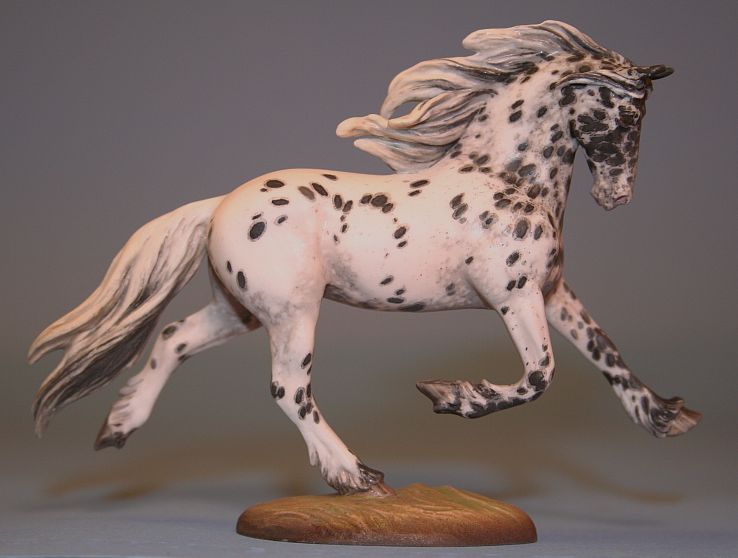This is an image of a strikingly detailed sculpture of a galloping horse, which appears to be either crafted from wood or painted ceramic. The horse is predominantly white, adorned with numerous black spots reminiscent of a Dalmatian. The sculpture captures the horse in mid-gallop, with its right rear hoof firmly planted on a round, medium-brown wooden base about the size of a man's hand, providing balance. The remaining legs are depicted in dynamic motion, emphasizing the speed and grace of the animal. Its mane flows backward in a dramatic display, transitioning from white to grey strands, as does its bushy tail which extends outward and up. The horse's head is lowered with black eyes and ears perked up, contributing to the lifelike energy of the piece. The background of the photograph is grey and neutral, ensuring that the finely painted details of the sculpture stand out. The overall effect is a captivating portrayal of motion and vitality.